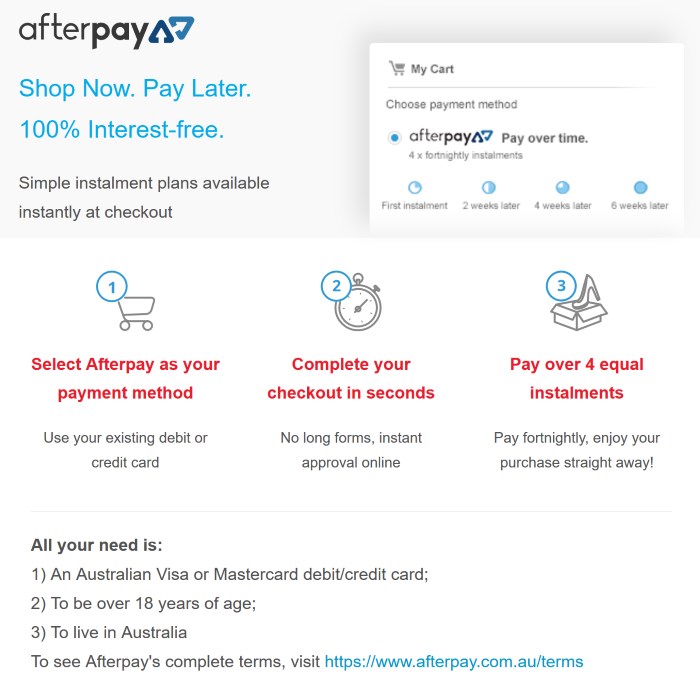The image is a detailed screenshot of a web page showcasing Afterpay's payment options. At the very top, there is a gray horizontal bar. On the top left-hand corner, the Afterpay logo is displayed with "After" in black text and "pay" in bold, accompanied by an icon of two triangles—one pointing up and the other pointing down. Below this, in medium blue font, the text reads: "Shop Now, Pay Later, 100% interest-free." This is followed by a note explaining that simple installment plans are available instantly at checkout.

On the right-hand side of the screenshot, there is a white rectangle containing the text "My Cart" and instructions to choose a payment method. It elaborates on the Afterpay option, which allows for payment over time through four fortnightly installments: the first installment is payable immediately, with subsequent installments due two, four, and six weeks later.

Underneath, further details are provided on how to use Afterpay: 
1. Select Afterpay as your payment method.
2. Use your existing debit or credit card.
3. Complete your checkout in seconds without needing to fill out long forms, since instant online approval is available.
4. Pay over four equal installments fortnightly.
5. Enjoy your purchase straight away.

At the top, from left to right, there are three icons accompanied by blue circles with numbers:
1. A shopping cart icon with a 1 in a blue circle.
2. A gray timer icon with a 2 in a blue circle.
3. A box with a high-heeled shoe sticking out of it and a 3 in a blue circle.

This descriptive caption provides a comprehensive view of the Afterpay payment process and its benefits as depicted in the screenshot.